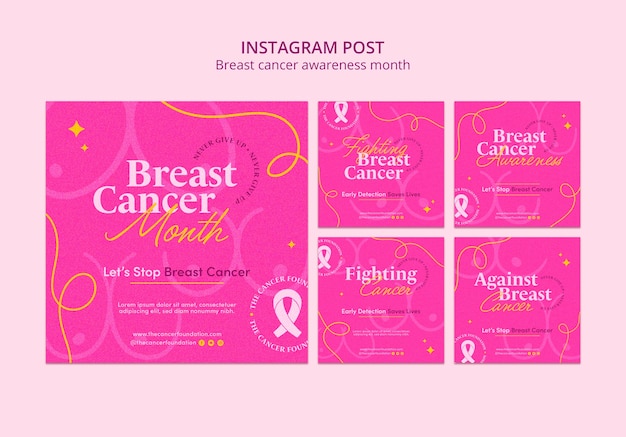This image is a screenshot of an Instagram post dedicated to Breast Cancer Awareness Month. The post features a large pale pink rectangle as the background. In the center, there are five bright pink boxes arranged with one large box on the left and four equally sized boxes on the right. The headline at the top, in a dark pink-purple color, reads "Breast Cancer Awareness Month."

Each of the bright pink boxes contains a slogan related to breast cancer awareness, accompanied by a pale pink looped ribbon, a symbol for breast cancer awareness. The slogans read:
1. "Breast Cancer Month"
2. "Let's Stop Breast Cancer"
3. "Fighting Breast Cancer"
4. "Breast Cancer Awareness"
5. "Against Breast Cancer"

These boxes and slogans are designed to promote awareness and highlight the importance of supporting those affected by breast cancer during the awareness month.